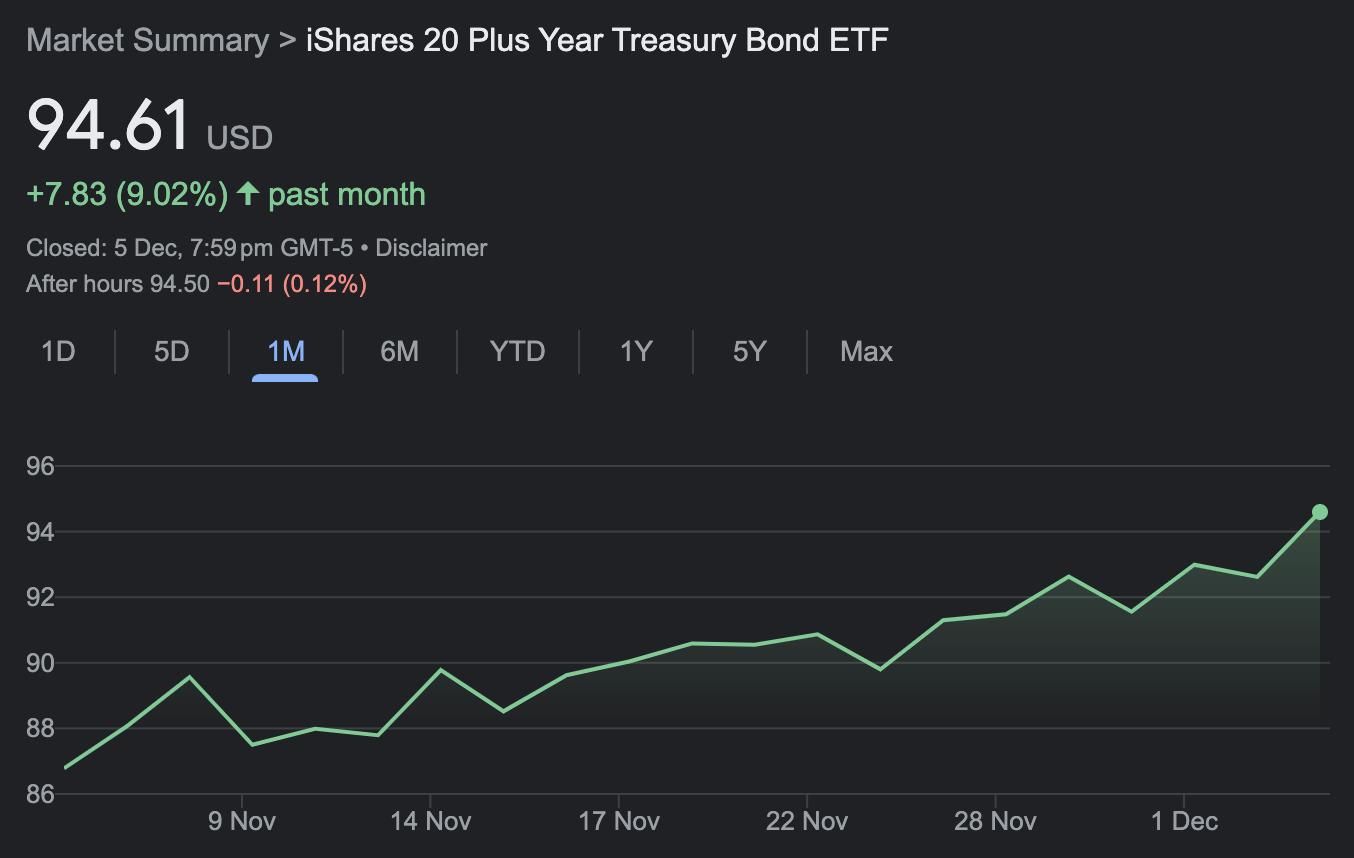The image depicts a Google stock summary in dark mode, characterized by a black background. In the top left corner, light gray text reads "Market Summary," followed by a right-pointing arrow. The stock being presented is the "iShares 20+ Year Treasury Bond ETF," highlighted in white text. 

On the left side, the current stock value is prominently displayed as "94.61 USD," with "USD" in light gray. Beneath this, the recent change in value is shown in green: "+7.83 (9.02%)," accompanied by an upward arrow indicating growth over the past month.

In a smaller font, a status update reads, "Closed 5 December, 7:59 PM GMT-5," followed by "Disclaimer" in light gray. Directly below, after-hours trading information is presented: "94.50," and it's noted in red text to have decreased by "-0.11 (0.12%)." 

Options for viewing the stock's performance over different periods are displayed from left to right: "1D, 5D, 1M, 6M, YTD, 1Y, 5Y, Max." The "1M" (one-month) option is highlighted in blue, indicating it is currently selected, while the other periods are in gray.

The stock graph, shown in green to signify an upward trend, traces the stock's performance from November to December. The graph starts at approximately 87 and climbs "scraggly" up to 95 by the end of the month, illustrating a clear upward trajectory.